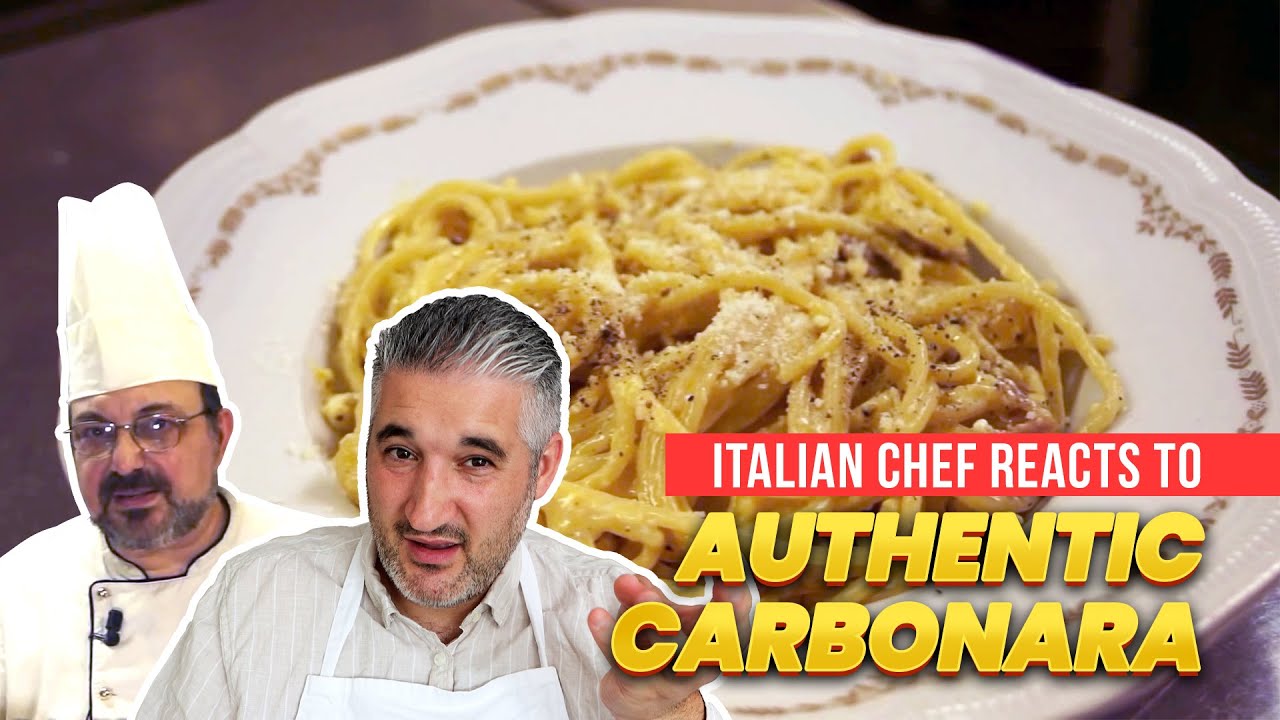In this image, we see an advertisement featuring two chefs situated in the bottom left corner, and a magnified dish in the background. The chef on the left is adorned in a classic white chef hat and uniform, complete with clear glasses and a grey and black beard. The chef on the right, sporting a grey collared shirt under a white apron, has gray and black hair and a thin beard. He appears to be gesturing, possibly making a point, while the chef with the hat remains expressionless. The background showcases a white plate with a golden-brown border, filled with what seems to be authentic carbonara—spaghetti noodles topped with Parmesan cheese and spices. The text overlay includes "Italian Chef Reacts to" in white letters on a red rectangle across the plate, and "Authentic Carbonara" in large yellow capital letters. The scene is set on a brown table, highlighting the appetizing pasta dish.